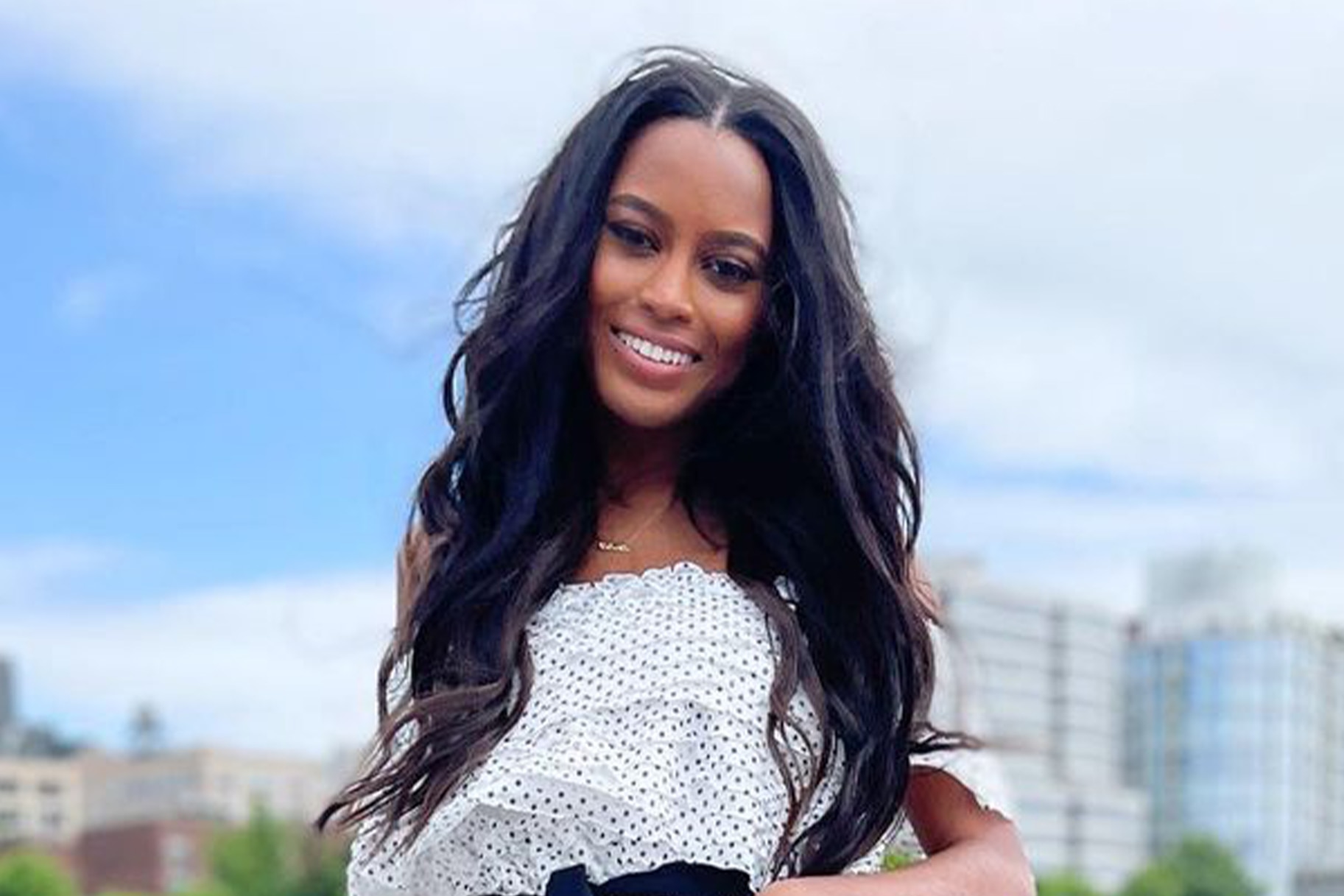The image features a young African American woman, likely in her early 20s, who is outdoors. She has long, slightly wavy black hair that cascades down her shoulders. Her complexion is dark yet radiant, and she has a slight, warm smile showcasing her white teeth as she looks directly at the camera. The woman is adorned with a gold necklace and is wearing a white, flowy blouse with multi-colored polka dots, predominantly blue. Her attire suggests a hint of a black belt around her waist. The background features a partly cloudy sky with patches of blue and an out-of-focus cityscape, including a mix of taller office buildings and shorter apartment structures. The blurred backdrop reveals some green treetops in front of the city buildings, adding depth to the urban scene.